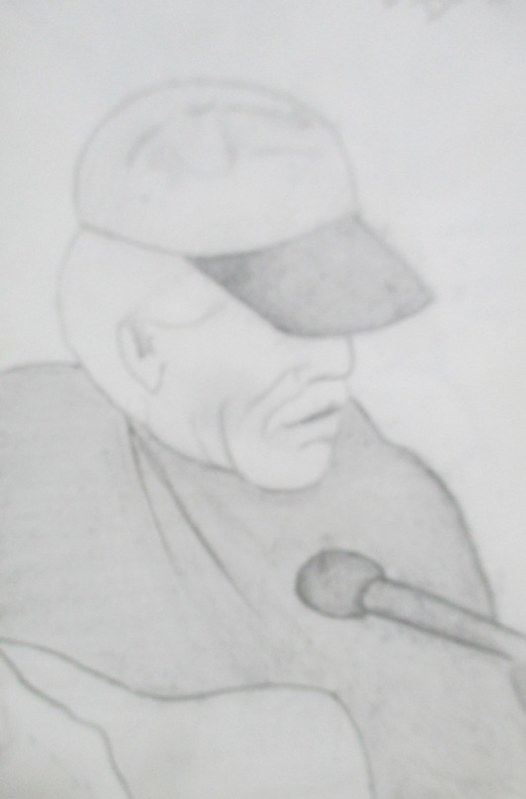A detailed sketch portrays an elderly man sporting a gray sweater. Positioned to his right, a microphone extends just below his chin, indicating he's likely speaking or singing. The man is characterized by a distinctive mustache, deep wrinkles etched across his cheeks, neck, and chin, and indistinct ears. His white hair is neatly tucked under a bald cap with a white crown and a black brim that sits low over his eyes. The man appears to be holding an object that resembles either a guitar or a balance board for a walker, adding an element of intrigue to the scene.